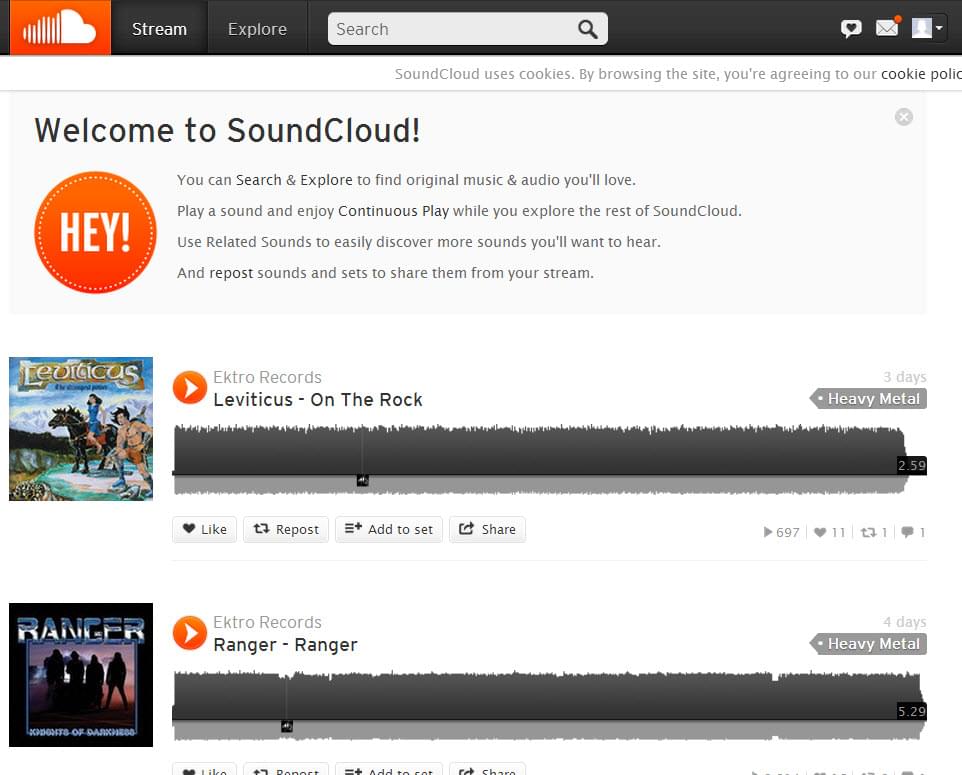The webpage displayed is SoundCloud, featuring the recognizable logo at the top—a rectangular orange background with a puffy white cloud partially comprised of horizontal lines on the left side. Visitors to the site are greeted by a message that explains SoundCloud's cookie policy, stating that by browsing the site, users agree to the use of cookies.

Below this, the page prominently includes a welcoming message: "Welcome to SoundCloud." An eye-catching orange button with an enthusiastic "Hey!" invites users to search and explore the platform for original music and audio they will love. It encourages them to play a sound and enjoy continuous play while browsing, using related sounds to discover more content easily. Users are also prompted to repost sounds and sets to share them from their own stream.

The page features two heavy metal tracks prominently. The first track is "On the Rock" by Leviticus, which includes an animated cover image. This is likely created by a familiar animation group. Users have options to play, like, repost, add to a set, or share this track. The second track is "Ranger" by Ectro Records, also a heavy metal song, suggesting a preference for this genre.

Overall, the webpage layout is user-friendly, encouraging exploration and interaction with the wide array of musical content available on SoundCloud.